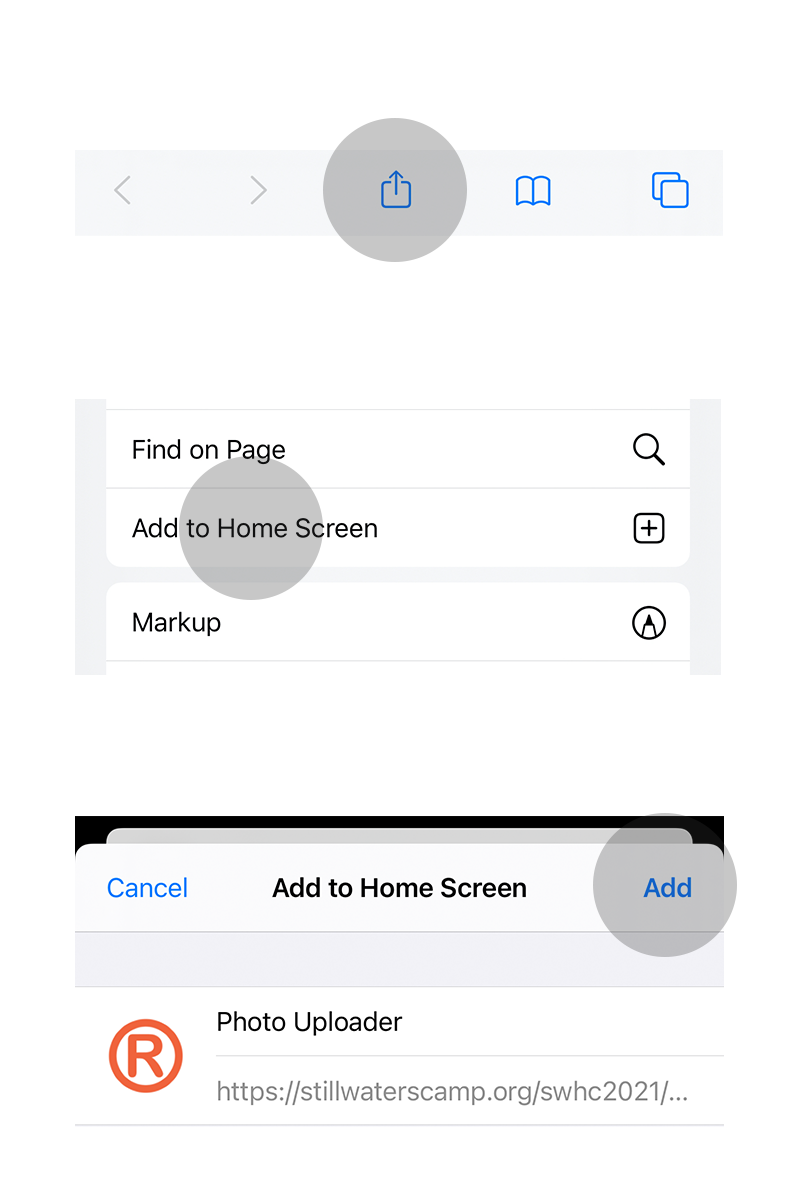The image depicts a settings menu, typically seen in a mobile browsing environment. At the top, there is a gray navigation bar featuring back and forward buttons, an open book icon, and a stacked square icon. 

Beneath this bar, there's a section showcasing different options: 
1. A square icon with a line through it and an upward arrow, encircled in gray.
2. A white section containing additional options: 
   - "Find on Page" accompanied by a magnifying glass icon.
   - "Add to Home Screen" represented by a square icon with a plus sign, which is highlighted by a gray circle.
   - "Mark Up" denoted by a circle with a pen tip icon.

At the bottom, the menu offers an action bar with a blue "Cancel" option to the left and a blue "Add" button to the right, also encircled in gray. 

Below this menu, there is a URL that reads "Photo Uploader, https://stillwatercamp.org/swhc2021/..." indicating a link to an educational resource, possibly for uploading photos.

The instructions seem to guide users to navigate to this URL and then add the photo uploader to their home screen using the provided menu options.